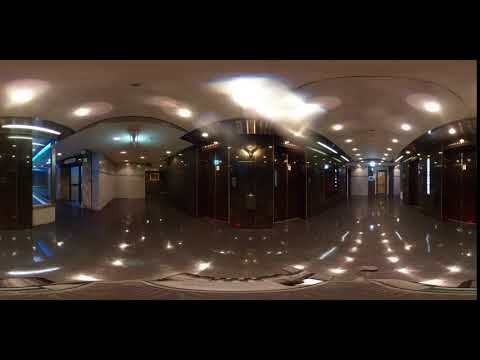The image depicts the interior of an elaborate, empty lobby, possibly within a fancy, older building such as the Empire State Building, showcasing a slight Art Deco style. This panoramic shot captures multiple perspectives, creating a rounded distortion that allows for a comprehensive view of the space. The walls are predominantly dark, either a deep brown or black, while the white ceiling sports curved molding, giving an impression of an arched design. The lobby is lit by numerous lights that vividly reflect off the glossy, gray marble-like floors, imbuing a sense of cleanliness and opulence. This polished floor extends into various hallways, punctuated by several doors leading to other rooms, and includes an elevator bank. Notably, blue LED lights illuminate one section of the image. The far left features a pathway leading to what appears to be a main glass exit door. The atmosphere is eerily quiet, as the space is devoid of people, yet fully lit, highlighting every detail.